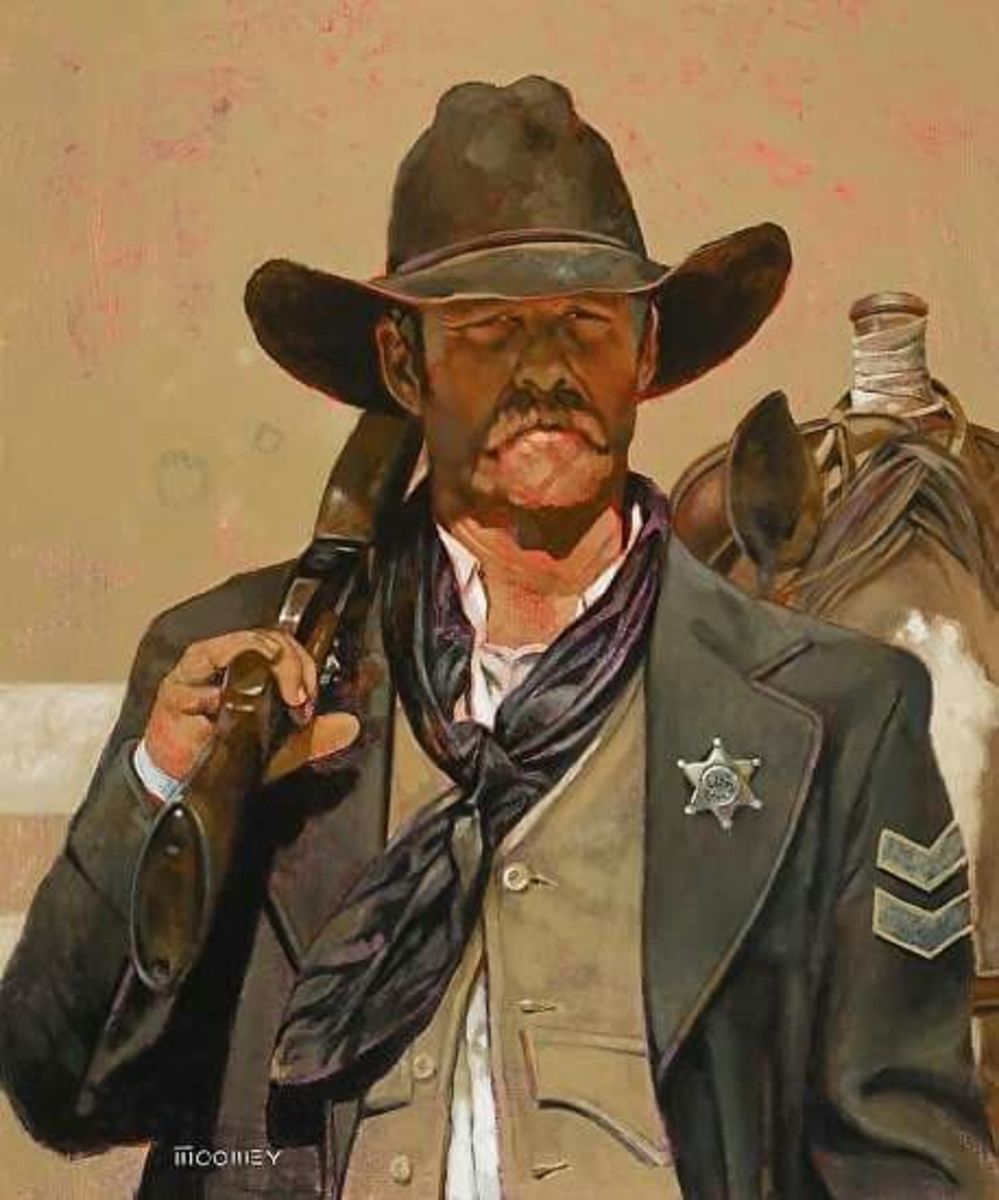This is a highly detailed and realistic painting of an Old West sheriff standing resolutely in the middle of a dusty street, his posture exuding authority. The sheriff, characterized by a weathered, serious expression, sports a dark brown Stetson hat and a prominent handlebar mustache. His piercing eyes seem to squint slightly as he gazes into the distance. Draped over his shoulder is a shotgun, its butt angled towards the viewer. He wears a distinctive dark blue Union War coat, signaling his past as a soldier, with a sheriff's badge pinned prominently on his lapel. Beneath the coat, the sheriff is attired in a light brown leather vest over a pristine white button-up shirt. Around his neck is a dark purple scarf, adding a touch of color to his rugged appearance. Behind him stands a faithfully saddled horse, identifiable by its brown ear, mane, and a white spot adorning its forehead. In the background, a fence runs alongside his right shoulder, subtly anchoring the scene in its historical context.